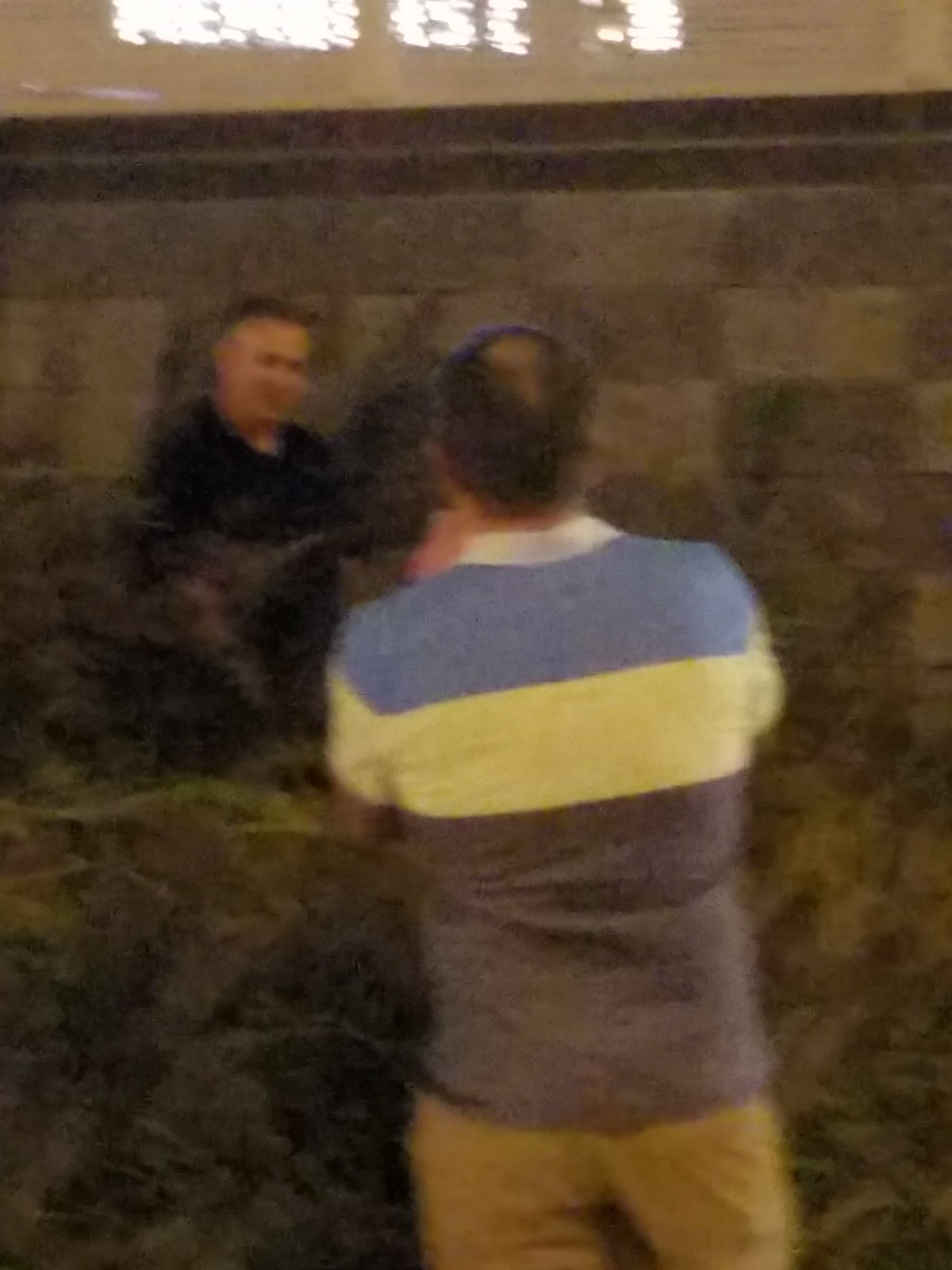A slightly blurry photo captures an intriguing scene involving two men separated by a lush green bush. The man seen from behind is wearing khaki pants and a tri-colored polo shirt featuring blue, white, and darker blue sections. His hair is short, predominantly dark with a distinctive bald spot shaped like an upside-down raindrop. It appears he might be holding a phone, potentially taking a photo or a selfie. Opposite him, the second man stands by a stone wall, donned in a black shirt or jacket. His hair is short with noticeable gray at the temples, and he seems to be smiling or engaging with the first man. Above them, a string of white lights forms words that are unclear in the photo, reminiscent of a stock ticker or decorative sign. The environment suggests an area resembling a customer service counter or a store display, adding to the scene's vibrant yet enigmatic ambiance.